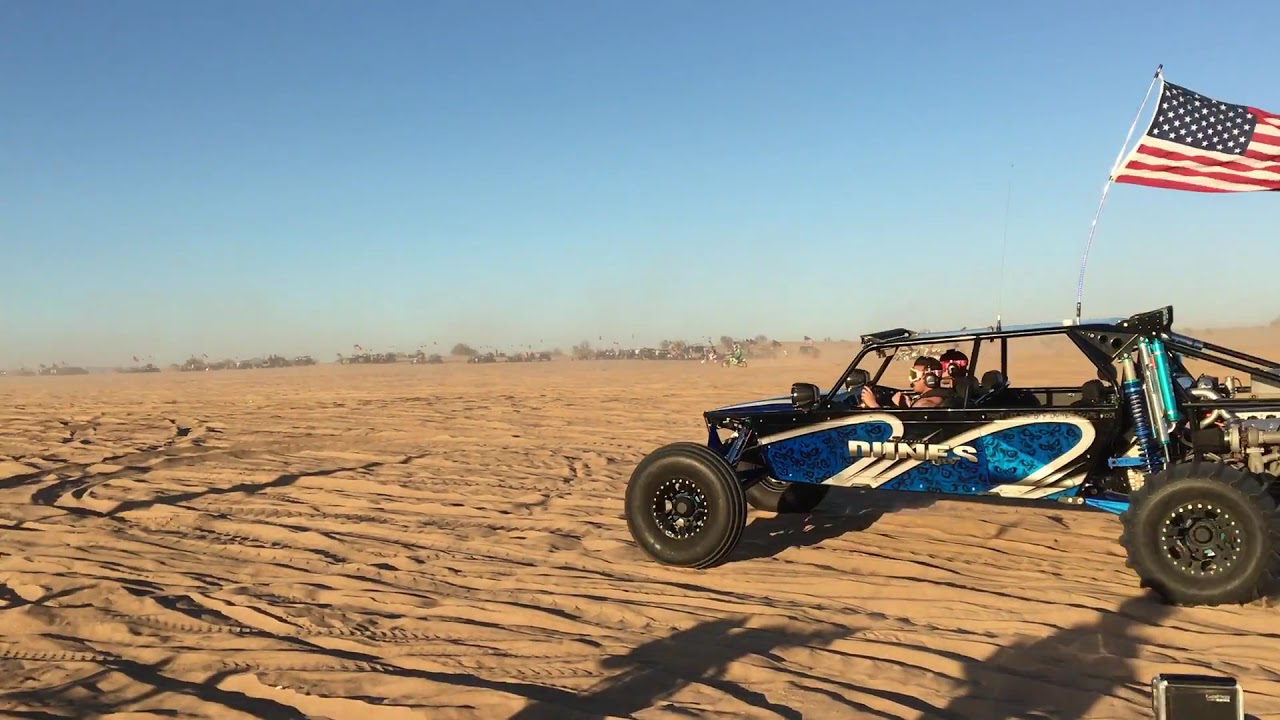The image captures a scene set in a bright, sandy environment reminiscent of a desert or sand dunes under a clear blue sky. Dominating the foreground is a striking blue and silver sand dune vehicle, adorned with blue shocks and suspension, and driven by two passengers sporting goggles and earmuffs. The vehicle is characterized by curved silver arches on its sides, with the word "Dunes" emblazoned prominently in bold, white uppercase letters with a gray drop shadow. This dynamic buggy features a black round tube frame, black spotlights, and black tires kicking up the dust as it carves through the beige sand, which is marked by many tire tracks. Attached to the vehicle is a long pole flying an American flag, vividly displaying its navy blue rectangle filled with white stars, and red and white horizontal stripes. In the far distance, a few buildings are faintly visible, while dirt bikes and other riders add to the adventurous atmosphere, suggesting a casual yet thrilling day of off-road fun. The entire setting is bathed in natural light, highlighting the vibrant colors and the energetic feel of the scene.